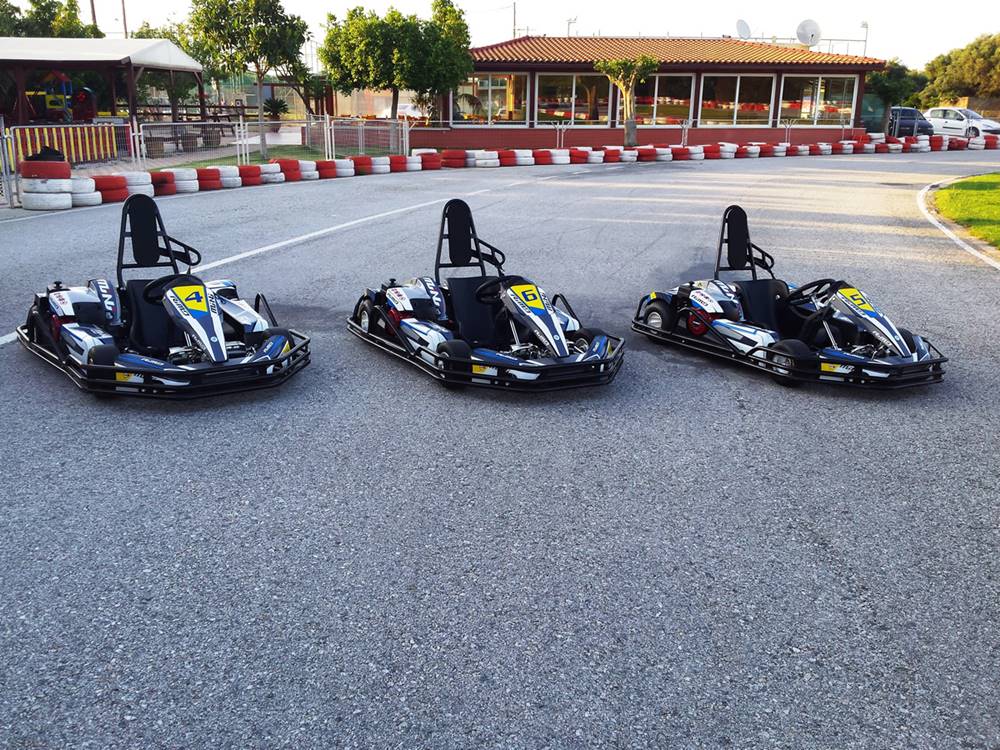This photograph showcases three empty go-karts lined up side by side in the middle of a smooth, medium-gray asphalt go-kart track. The karts, which are black with white and blue highlights, are identified by the blue numbers 4, 5, and 6 on a yellow background. They are positioned diagonally from left to right, giving a dynamic view of their sleek, fast design. Surrounding the track are red and white tires acting as safety barriers stretching into the distance. In the background, there are some buildings, likely facilities for track entry and services, along with a small parking lot that has a couple of real cars parked. The scene is set outdoors, under daylight, with trees adding a touch of greenery beyond the fence that encloses the track area.